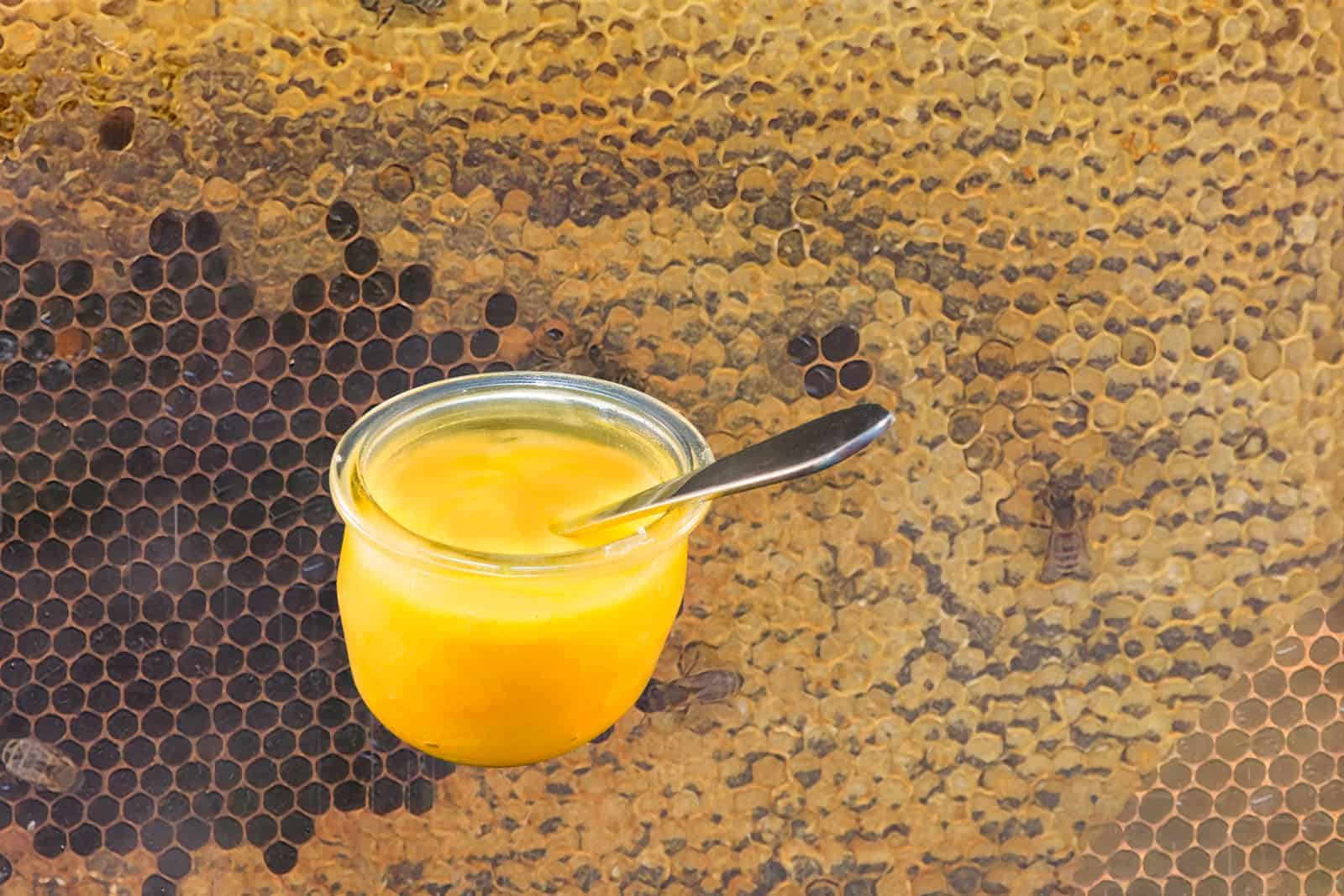In the image, a small glass jar brimming with a rich yellow-gold liquid, likely honey, sits prominently on top of honeycombs. The jar, which has no lid and features a lip at the top, has a piece of silverware submerged within it, with its handle sticking out. Surrounding the jar, the honeycombs, which form the background of the image, showcase differing states; some are black and seemingly emptied, especially to the left, while others are filled with substances ranging from yellowish to dark brown. Several bees can be seen hovering around the scene, emphasizing the connection between the honey in the jar and its origin from the beehive. The vibrant color of the honey and the presence of the bees work together to clearly showcase the natural source of the honey.